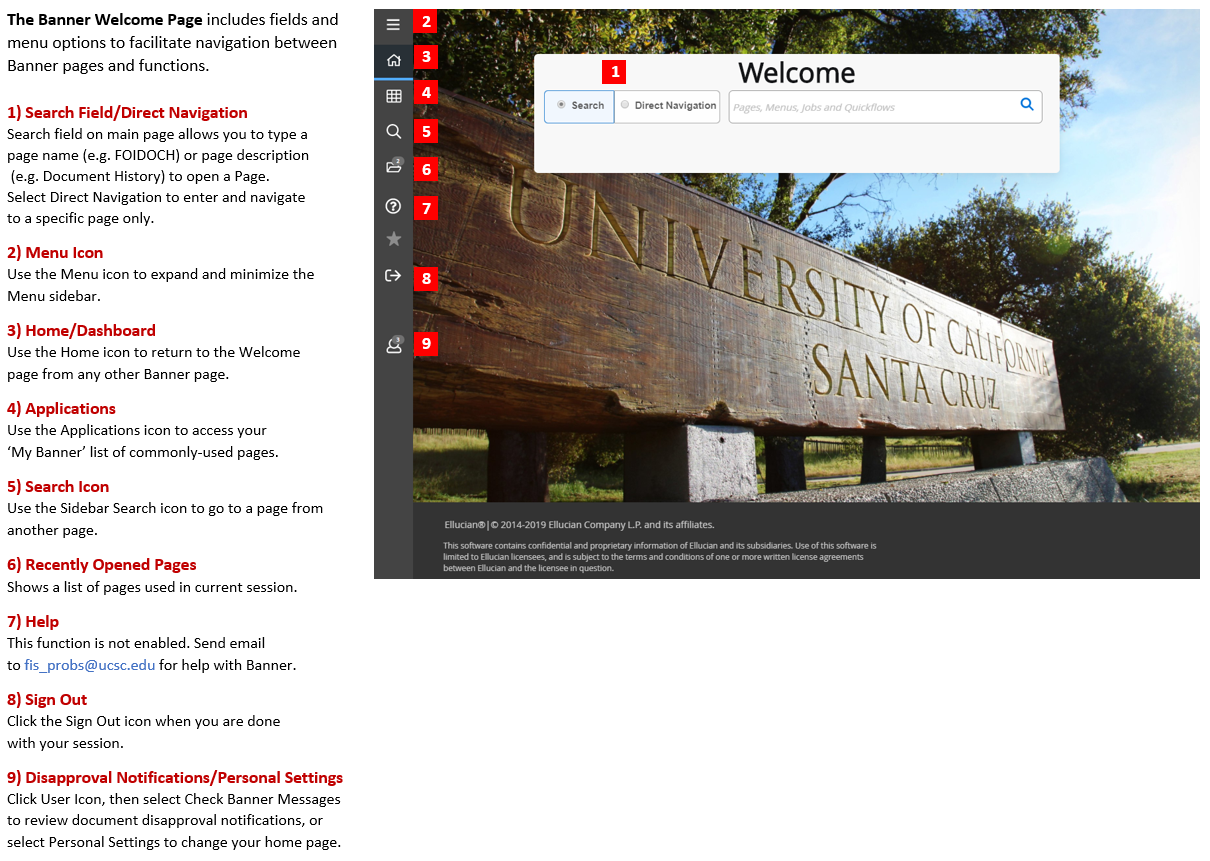The screenshot features a webpage with a dual-pane layout. On the left side, information is listed vertically, while the right side includes a navigation area, search bar, and a welcoming message. The webpage prominently displays an image of a wooden sign reading "University of California Santa Cruz," set against a backdrop of trees and a vibrant blue sky, with a stone landscape in the foreground.

Details on the right side of the page include:
- A navigation menu and search area at the top.
- A banner welcome page providing fields and menu options to facilitate easy navigation between different sections, indicated in red text. 
  - Menu options include: Home Dashboard, Application, Search Icon, Recently Opened Pages, Help, Sign Out, Disapproval Notifications, and Personal Settings, each accompanied by descriptive black text below.
  
Below the search bar and navigation links are cubicle-style sections, including the home page, search page, and folders for better organization.

The intuitive design, with organized menu options and clear labels, ensures users can efficiently navigate the University of California Santa Cruz's online resources. The welcome page is clean, featuring a white background, easy-to-read text, and numbered sections for straightforward navigation.